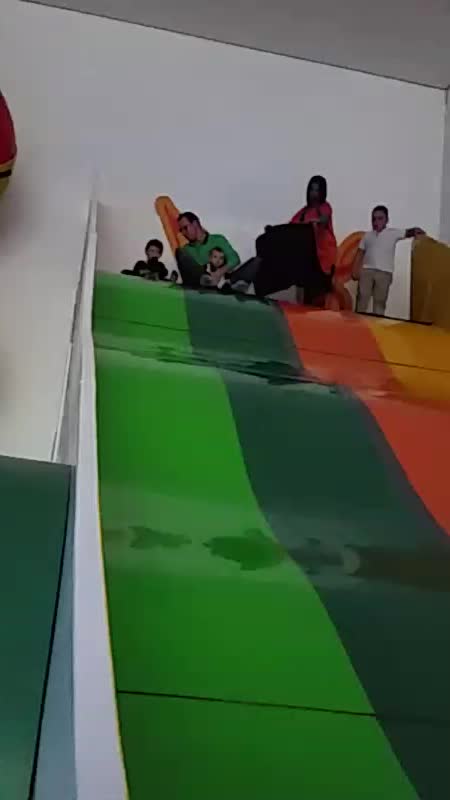The photograph captures a large, multicolored sliding board towering up to 30 or 40 feet high, situated against a white wall and ceiling in an indoor area. This massive slide, featuring rolling wave-like bumps, is divided into multiple lanes colored light green, dark green, orange, and yellow. At the top of the slide, several people are preparing to descend, using mats for the ride. Among them are a man wearing a green sweater holding a toddler in a green shirt, a little boy in a white shirt, a girl in an orange shirt with a black mat, and a person in a red shirt. The scene is lively with anticipation as these individuals sit and stand, ready to experience the thrilling descent.